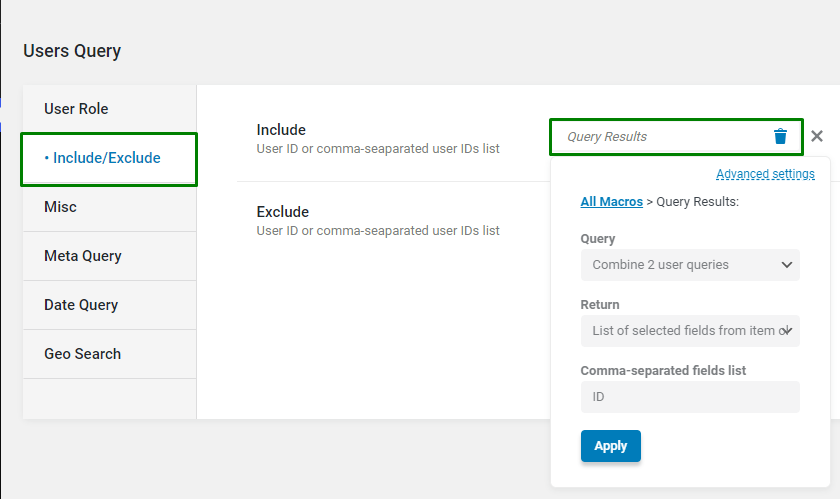This image showcases the user's query interface within a software application. The interface is presented in a square format featuring a settings menu against a grayish background. On the left side of the screen, there's a vertical menu, prominently located in the upper left corner. The menu items include:

1. **Include/Exclude:** Highlighted in a blue font and surrounded by a green square border.
2. **MIS:** Listed directly below the Include/Exclude option.
3. **Meta Query:** Following the MIS option.
4. **Day Query:** Positioned beneath the Meta Query option.
5. **Geo Search:** The last item on the list.

To the right of this vertical menu, the include and exclude options are stacked above each other. Further to the right, enclosed within a green square outline, is the section for "Query Results," which bears a blue trashcan symbol. Below this segment is the area for "Advanced Settings," which details options such as "All Macros," "Query Return," and "Comma-Separated Fields List."

The interface is designed to provide users with organized and easily accessible query management options, enhancing their operational efficiency.